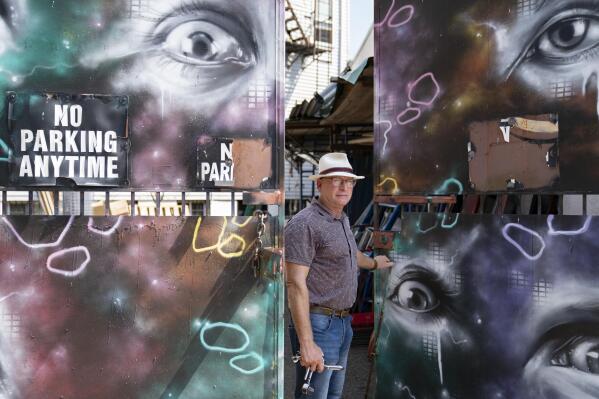The photograph captures a 50-something white man wearing glasses, a white hat, and a tucked-in grey polo shirt paired with blue jeans and a brown belt. He stands just inside a metallic gate, looking outward towards the viewer. The gate itself is a vivid piece of digital artwork, painted with striking details: a set of huge, terrified eyes on the left, a neutral eye on the right, and two more fearful eyes at the bottom. The gate also bears the bold text: "No Parking Anytime," creating the impression that these eyes are watching you, reinforcing the message. The artwork is further accentuated with muted shades of purple, blue, and green, creating a surreal and somewhat eerie atmosphere. In the background stands a white two-story building with a fire escape, adding an urban context to this intriguing scene.